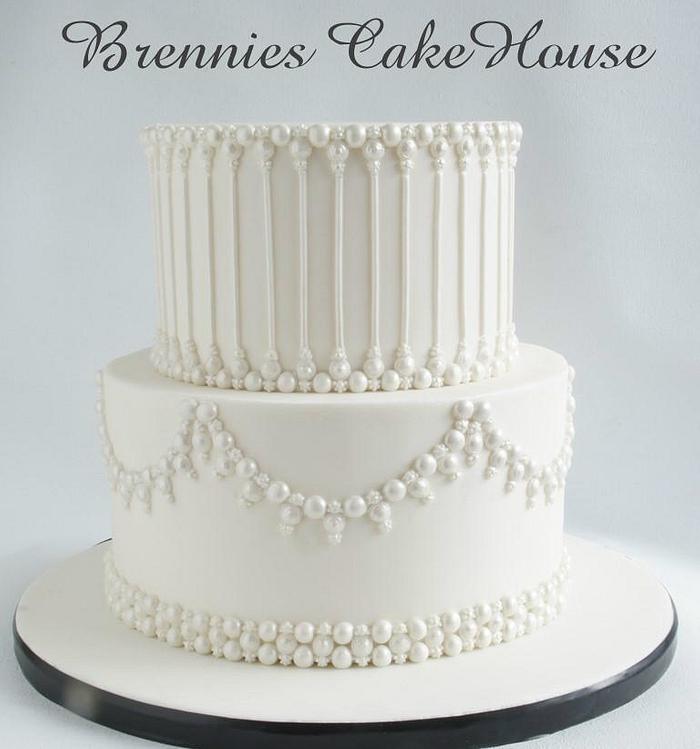In the center of the image stands a pristine wedding cake, set on a white base plate that is bordered with black. The cake features two round cylindrical layers, both entirely white. The larger bottom layer is adorned with a neatly arranged row of beads resembling delicate pearl necklaces, with additional bead arches providing elegant decoration. The smaller top layer, which sits atop the base, includes a series of columns encircling it, also fashioned from beads. White beads embellish both the top and bottom edges of this upper tier. Crowning the cake is a black text inscription that reads, "Brenny's Cake House," completing the refined and sophisticated design. The background is light blue, accentuating the stark contrast of the cake against its setting.